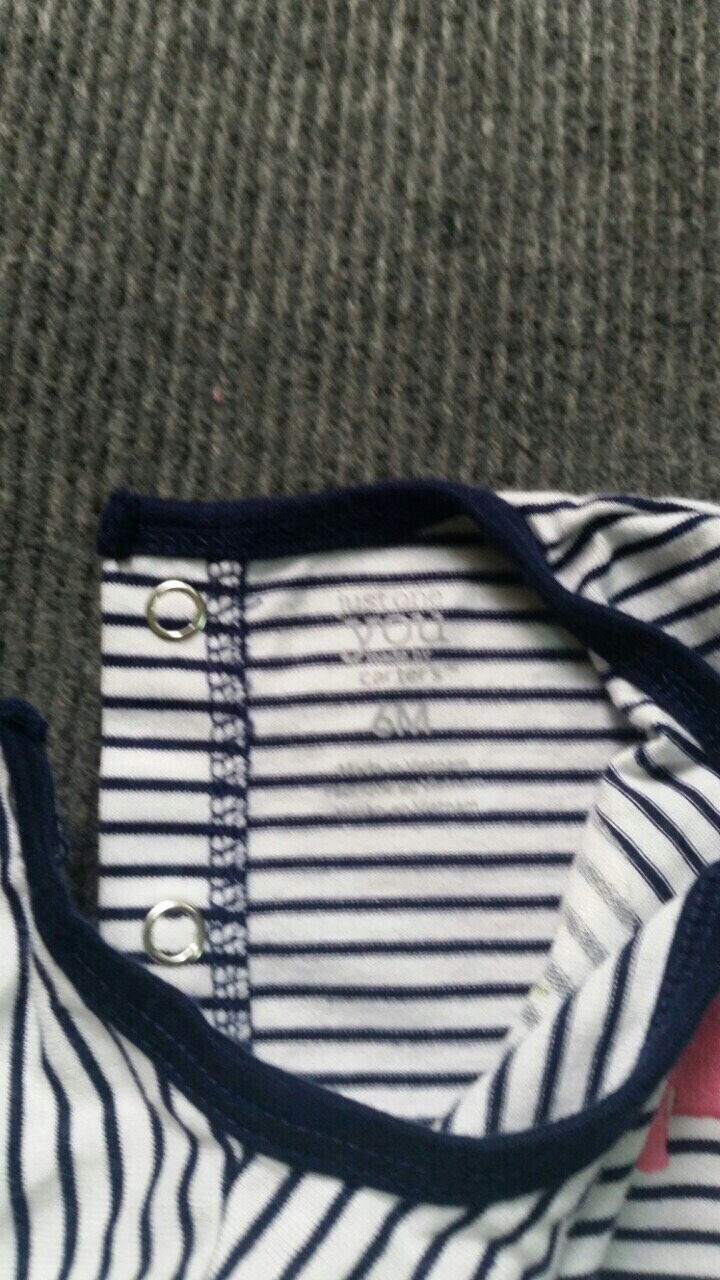The image captures a scene featuring a carpeted floor in a dark gray shade, interspersed with lighter gray vertical lines. On top of this patterned carpet lies a shirt, predominantly colored in dark blue and white. The hem of the shirt is a solid dark navy blue. The shirt features thin dark navy blue horizontal stripes alternating with thicker white horizontal stripes, creating a visually appealing pattern. The vertical lines of the shirt pattern can be observed near the sleeve areas, maintaining the same navy blue and white striped design.